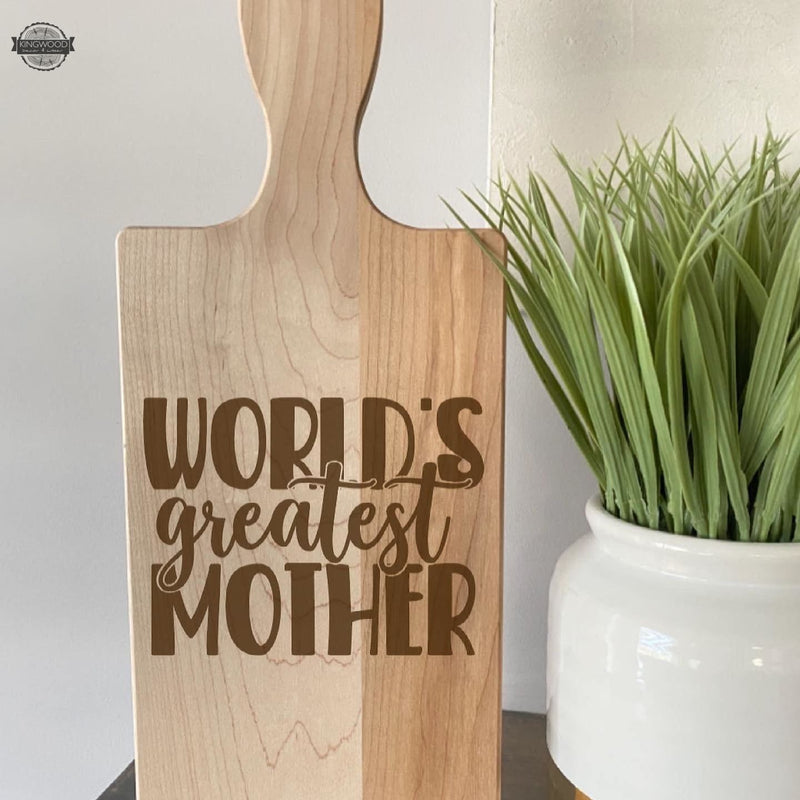In this detailed image, a wooden cutting board with a rectangular base and a handle on top sits prominently in the center. The board is divided into two parts: one part is light brown while the other is a medium brown shade. Written on the board in dark brown text are the words, "World's Greatest Mother," with "World's" and "Mother" capitalized and "greatest" in lowercase. To the right of the cutting board, there is a white flower pot adorned with a gold rim at the bottom, containing long, green leaves that resemble herbs. The board and pot rest on a brown table. In the background, the wall is mostly white, with a contrasting beige section. In the top left corner, a circular logo with the words "Kingswood" written in white letters on a black and grey background is visible. The setting appears to be inside a kitchen, with the simple yet charming décor creating a warm and welcoming atmosphere.